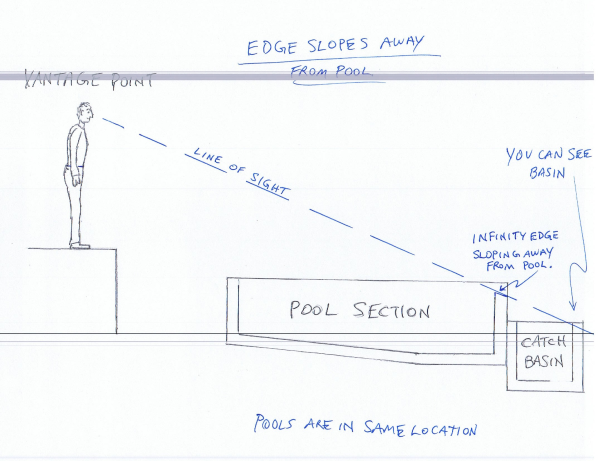The diagram is a detailed drawing illustrating how an infinity edge pool works. It features a black and white side view of a person, drawn almost like a stick figure but with clothing, standing on a ledge labeled "vantage point." From the person's vantage point, a dotted blue line labeled "line of sight" extends diagonally downward to the "pool section." The pool has an outer edge leading to a catch basin, both labeled in black text. At the top of the diagram, blue text underlined reads "edges slope away from pool." Along the back of the pool and catch basin, the text indicates "infinity edge sloping away from pool" and "you can see basin." At the bottom, a note in blue text confirms that "pools are in the same location." The diagram visually explains that water flows from the infinity edge of the pool into the catch basin, where it is likely recycled.